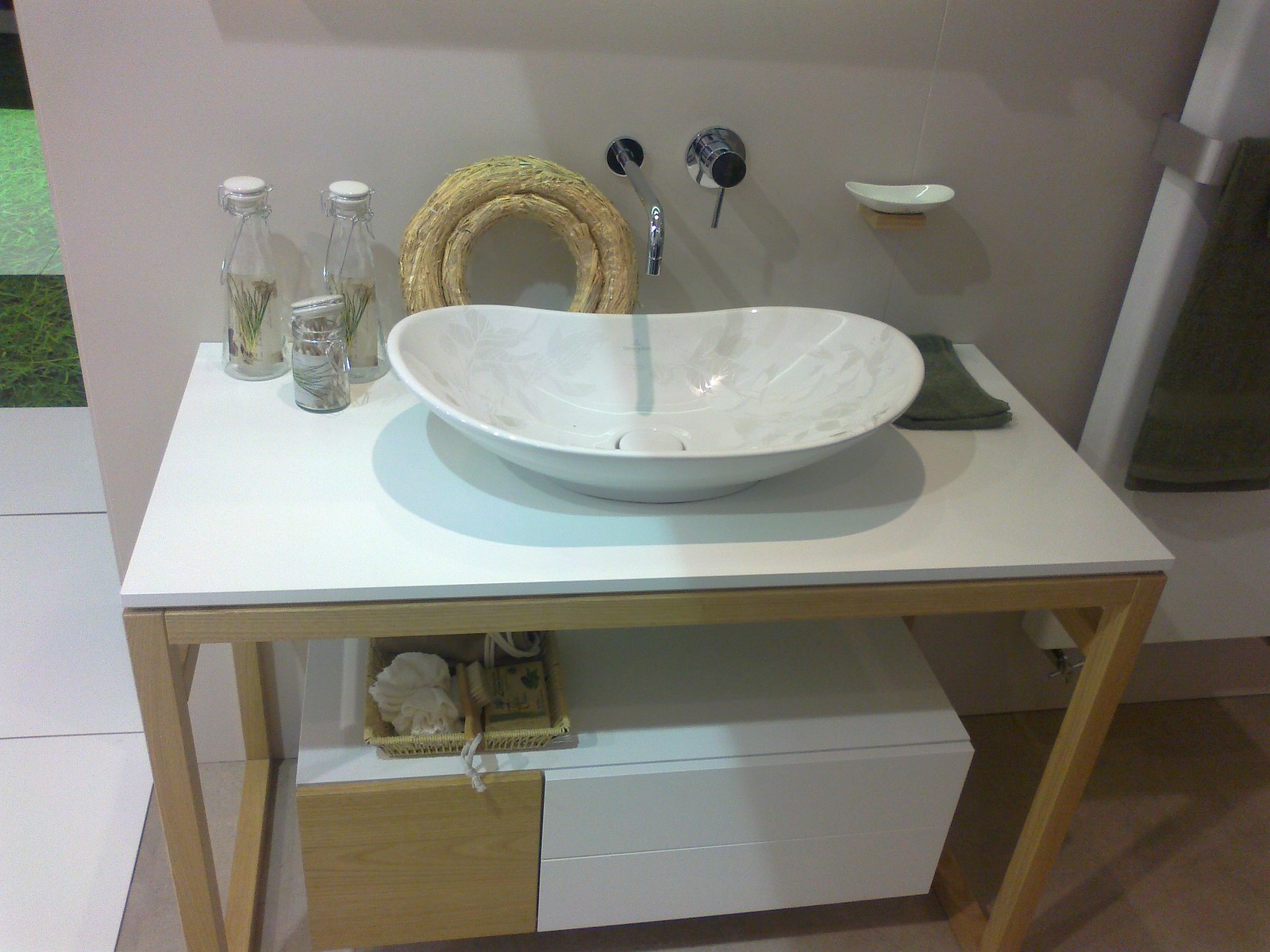This image showcases a meticulously designed mid-century modern bathroom sink setup. The elegant counter is supported by four minimalistic legs, which are connected at the bottom, forming two box-like structures on either side. Nestled beneath the counter is a stylish chest of drawers, featuring two long, slender, white drawers accented by natural wood, paired with a single square wooden drawer for additional storage. Atop these drawers sits an organized tray holding a bar of soap and a loofah sponge, emphasizing both functionality and aesthetic appeal. The counter itself is crafted from pristine white Formica, lending a sleek and clean look to the space. Complementing this setup are several decorative bottles filled with aromatic scents or spices, adorned with a few blades of grass, adding a touch of nature and sophistication. The sink is an oblong, oval-shaped basin with a white finish sprinkled with subtle gray granular tones. It features a singular, elegant faucet in the center, accompanied by a single handle to the right for easy water control. Additionally, an oval soap dish hangs gracefully from the wall, completing this beautifully designed bathroom arrangement.